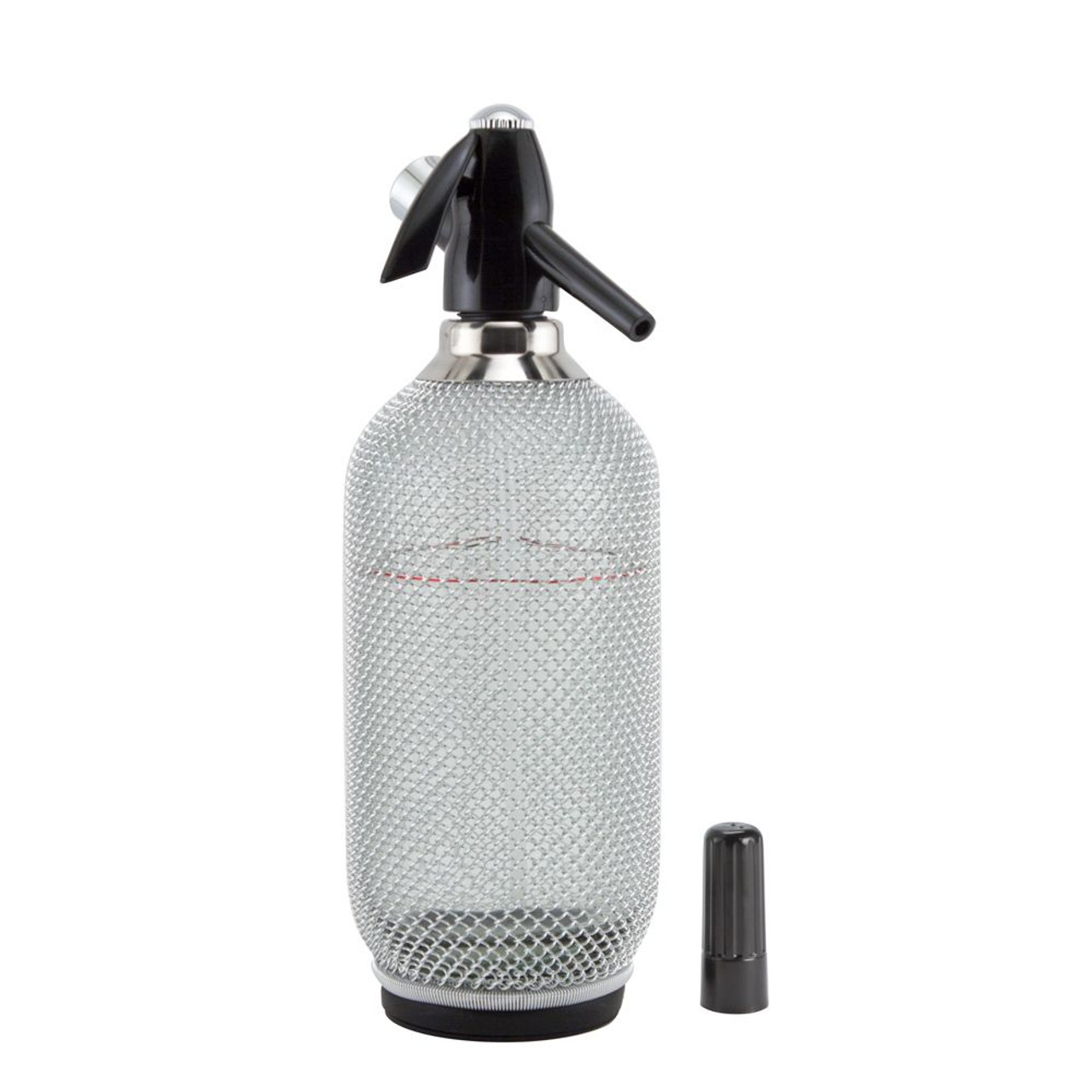This black and white photograph showcases a transparent canister that appears to be either plastic or glass with a rough, crystal-like texture on its outside. The canister, which strongly resembles a fire extinguisher or spray bottle, features a black base made of what looks like rubber or plastic. The top of the canister is adorned with a silver metal piece and transitions into a black section with a nozzle aimed downward, likely for dispensing liquid or air. This nozzle includes a turning button, or dial, which appears silver and is used to adjust the output. A black lid, which seems to cover the nozzle to prevent leakage, lies next to the canister on the right. The entire setup conveys a utilitarian design, blending both form and function.